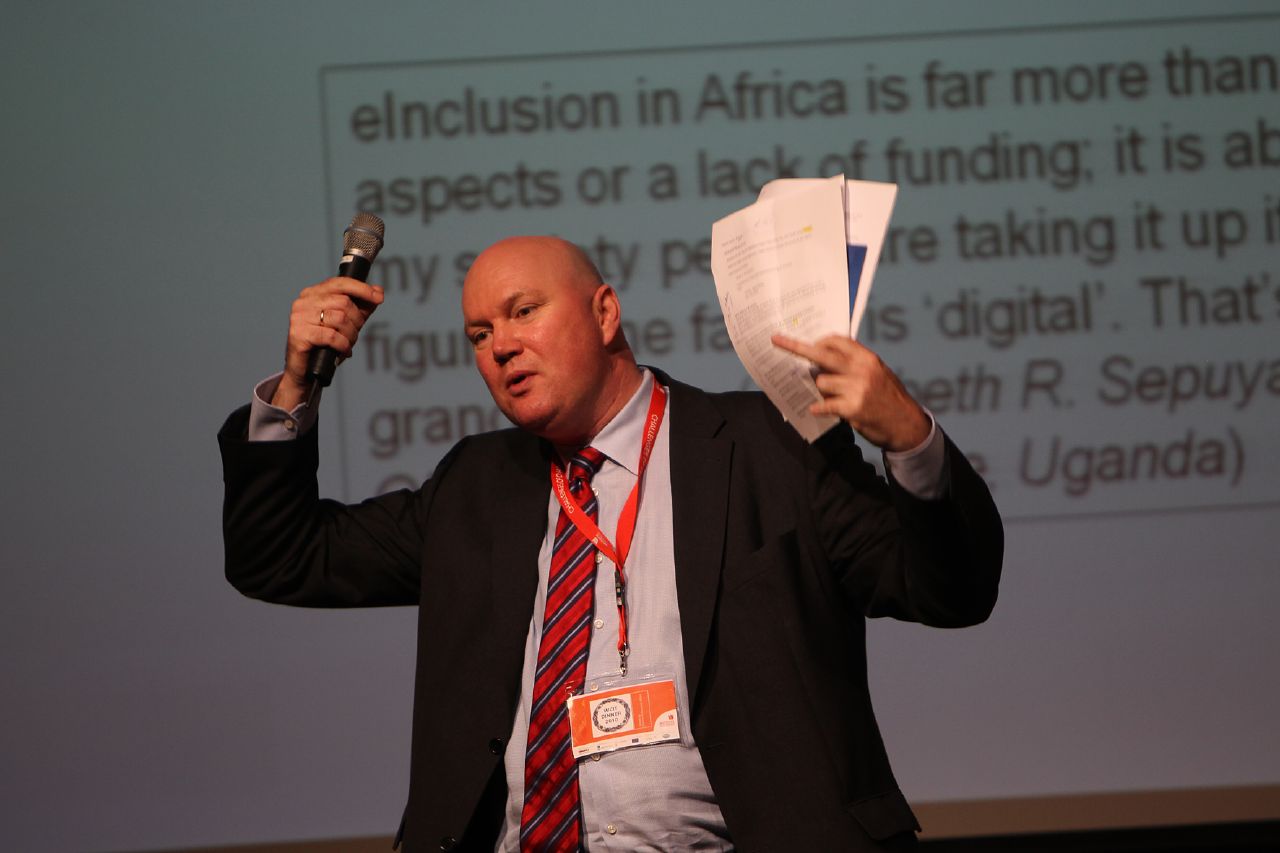The image depicts a formal presentation with a bald man, likely in his mid-40s to 50, standing on stage. He is dressed in a black suit paired with a light blue collared shirt and a red and blue tie. An orange lanyard with a pass is visibly hanging around his neck. In his right hand, he holds a microphone, while his left hand clutches two pieces of paper, possibly his speech transcript. Behind him, text from a PowerPoint slide is partially visible, reading, "inclusion in Africa is far more than aspects or lack of funding. It is...," with the remaining content obscured by his body. His mouth is open as if he is mid-sentence, and he appears to be intently engaging with the audience.